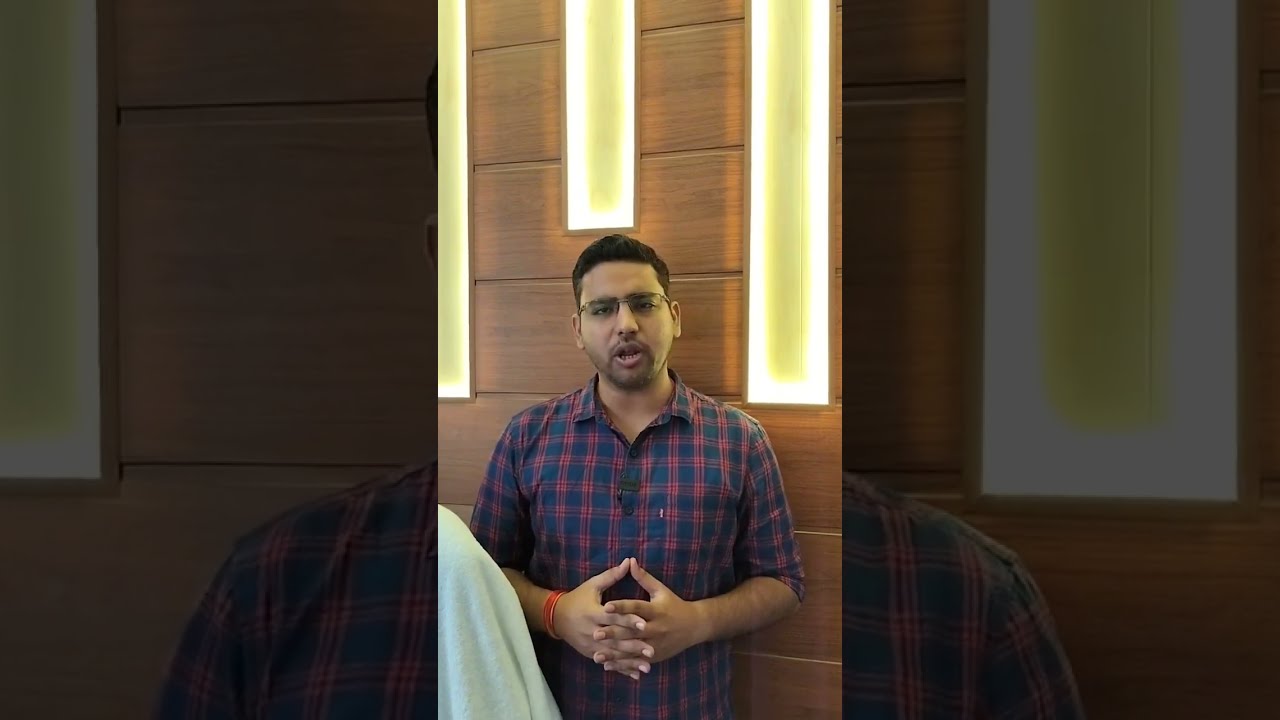In this image, a man in his early 30s stands centered against a background of light wood paneling. The wood wall behind him features three vertical lights: one directly above his head, and two slightly behind his shoulders, emitting a combination of yellow and white light. The man, who has short black hair, glasses, and stubble, wears a blue and red plaid short-sleeve button-down shirt. He also has an orange bracelet on his wrist, highlighting a distinct sunburn line where a watch used to be. His hands are clasped together in front of him at his abdomen. To his right, near his elbow, there appears to be a light blue inanimate object, possibly covered with a blanket. The setting suggests he is giving a speech or presentation.